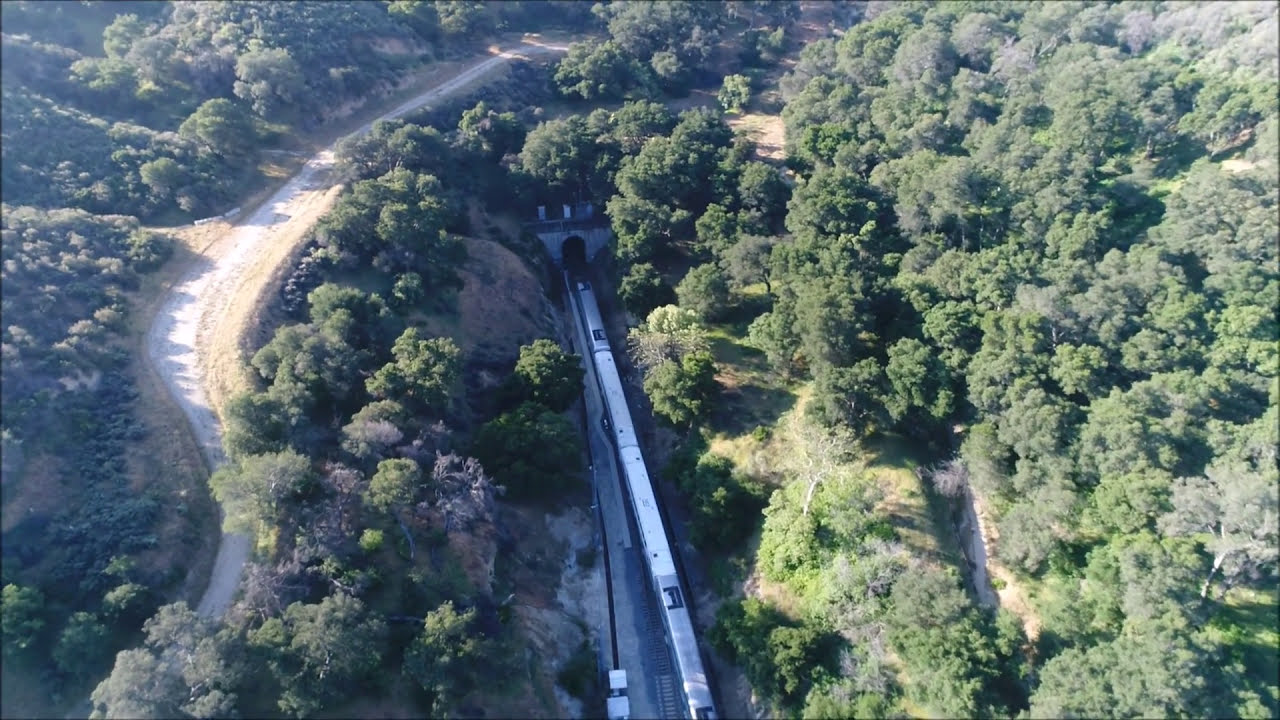An aerial view captures a scenic, wooded area dominated by vibrant green foliage, indicative of spring or summer. In the center of the image, a lengthy, shiny silver train, resembling an Amtrak, snakes its way through, nearly spanning the entire frame. The train is on the verge of entering a stone tunnel with a gray arch, which runs underneath a dirt-paved road. This road winds from the bottom left of the image up to beyond the top of the train's path. To the right of the train tracks, a hilly range is densely packed with a mix of light and dark green trees, bushes, and grassy areas. On the left, another hill dotted with trees and greenery features dirt paths snaking through the landscape. The scene is a picturesque blend of natural beauty and man-made infrastructure.